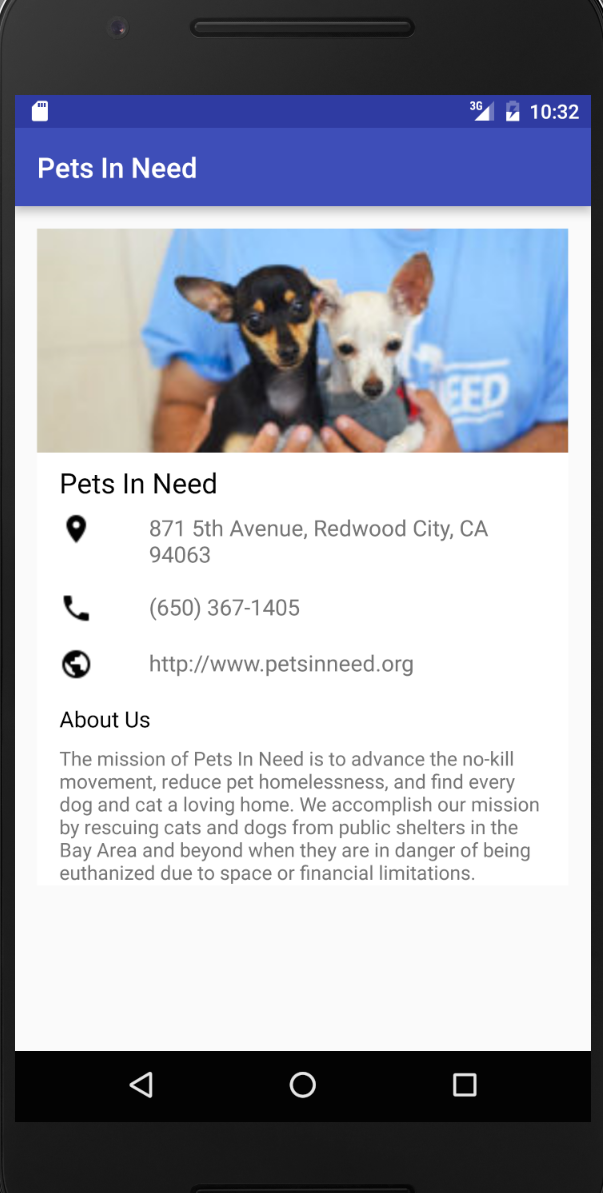The image depicts a web page being accessed on a mobile phone, as evidenced by several features in the top-right corner of the screen. Here, white icons indicate the phone's current status: a signal strength meter displaying 3G connectivity, a battery icon showing that the device is charging, and the time, which reads 10:32. This portion of the screen is accentuated with a navy-blue background.

In the top-left of this navy-blue area, white text reads "Pets In Need." Directly below is a prominent photograph of an individual wearing a blue shirt, holding two tiny chihuahuas—one is black and brown to the left, and the other is white to the right. The person's head is not visible; only their torso and hands, which are cradling the small dogs, are shown.

The lower portion of the webpage transitions to a white background, where the phrase "Pets In Need" appears again in black text. This section includes additional details such as an address, a phone number, a website URL, and an "About Us" message describing the mission and activities of the Pets In Need organization. This neatly structured layout effectively combines visual and textual elements to provide comprehensive information about the organization.